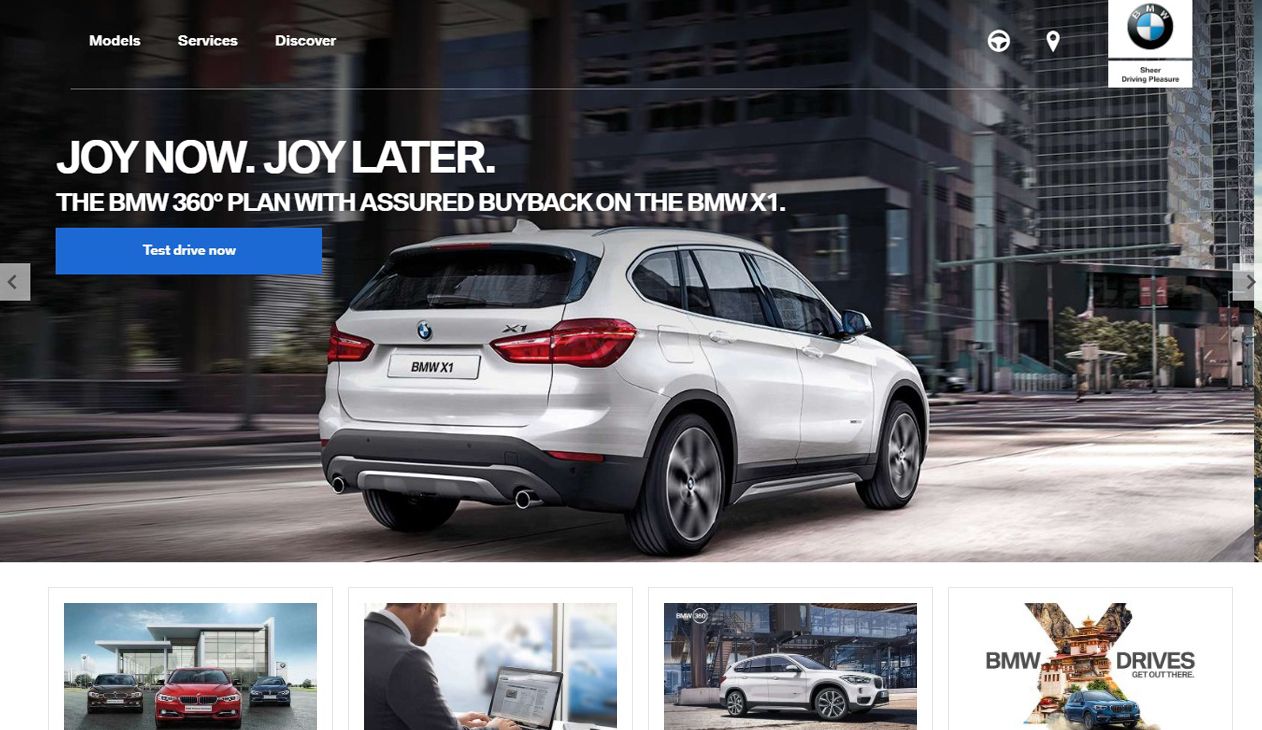The image appears to be a section of a BMW car company's website, meticulously designed with a clean and modern aesthetic. 

In the top right corner, the iconic BMW logo is prominently featured within a black circular background, with "BMW" emblazoned in crisp white text. On the opposite side, the navigation menu offers three options—Models, Services, and Discover—each elegantly displayed in white text on a transparent background.

Dominating the central portion of the page is a striking image of a light gray BMW X1, majestically driving to the right. The vehicle's license plate clearly reads "BMW X1," amplifying its brand identity. Above this visual, hovering in sleek white text, is the slogan "Joy Now, Joy Later. The BMW 360 plan with a shirt buyback on the BMW X1." This message conveys a sense of dual satisfaction—both immediate and future joy—accompanied by an innovative buyback program.

Directly below this statement, a vivid blue rectangle serves as a call-to-action button, urging visitors with the inviting words, "Test Drive Now," written in white.

Lastly, the bottom section of the image is divided into four distinct square boxes, each portraying different aspects of the BMW experience. 
- The first box showcases three BMW vehicles facing the viewer, with colors ranging from dark brown, to red, to black.
- The second box depicts a person engaged with a laptop, symbolizing online services or connectivity.
- The third box features a white SUV, highlighting another model in the BMW lineup.
- The fourth box, simply labeled "BMW Drives," suggests various driving experiences or programs offered by the company.